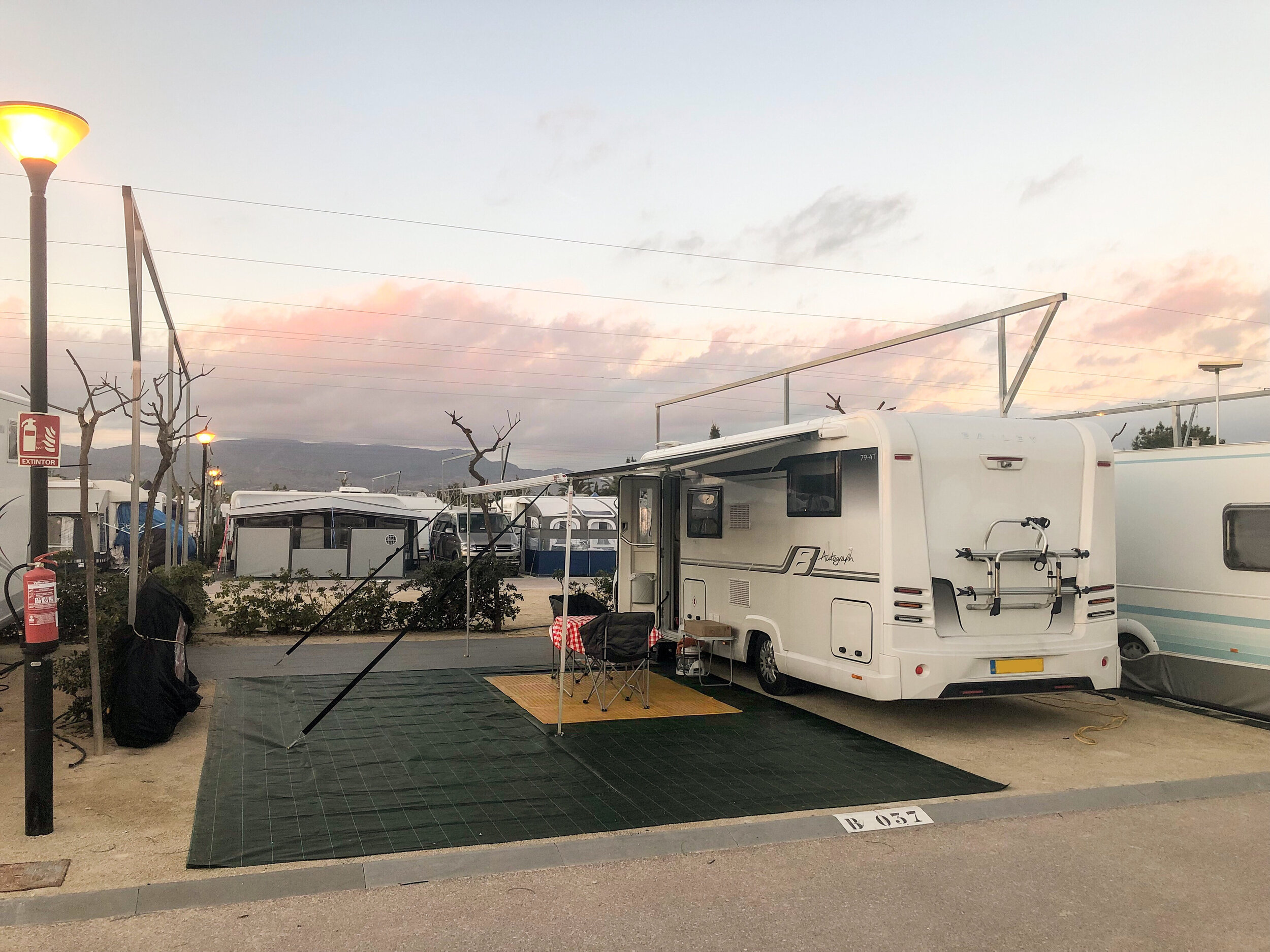The image depicts a vibrant RV lot captured during sunset, showcasing a scenic and organized setup. Centrally featured is an open RV lot with a prominently displayed black tarp underneath. An awning extends over the layout with a checkered red and white tablecloth covering a table and two black chairs set up for a meal. To the right of this setup is an RV with its doors open, and a portion of another RV is visible further to the right with more RVs receding into the background.

On the far left of the image, a black lamppost topped with a yellow light is seen, and attached to it is a fire extinguisher. Power lines run horizontally across the scene, contributing to the structured environment. Midway in the distant background, an imposing mountain range stretches across, under a partly cloudy sky accented with shades of pink, blue, and gray indicative of the setting sun. In the foreground, the concrete ground is clearly marked with the lot number "B037" in stark black on a white background. The scene vividly captures the organized yet serene atmosphere of the RV campground, blending natural beauty with a touch of everyday practicality.